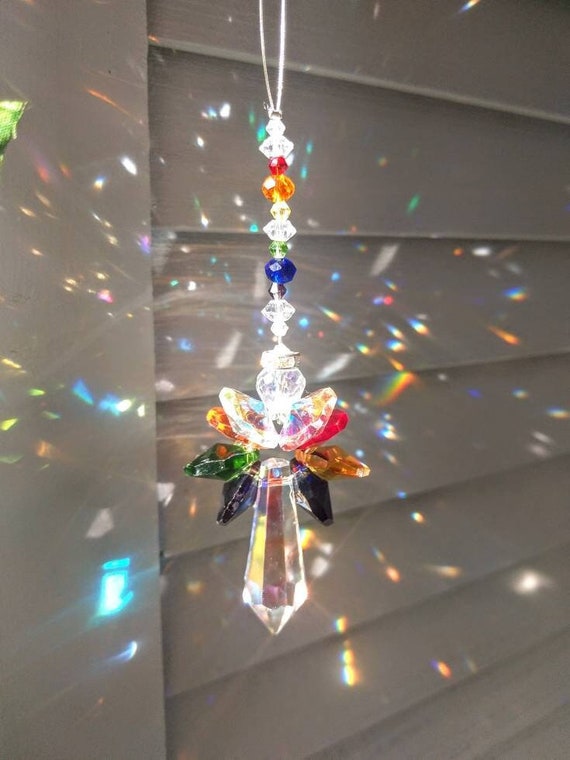This image features an intricately designed wind chime adorned with an array of vibrant crystals and beads, hanging gracefully from the ceiling or side of a white house with slatted siding or window cover. The wind chime is a mix of small, colorful beads—white, red, orange, green, blue, silver, and clear—that cascade down a thin line or chain. Toward the bottom, the crystals become larger and include shades of red, green, purple, pink, and orange. The design culminates in a prominent, clear, pointed crystal that forms the body of an angel, with a round crystal for the head and slender crystals serving as the wings.

The photo, taken during a sunny moment, captures the sunlight filtering through these multi-colored crystals, casting a dazzling array of red, yellow, blue, green, orange, and white reflections onto the background. These reflections create a vivid display of colors on the white siding, enhancing the visual appeal of the wind chime. The wind chime is centered in the image, highlighting its elaborate and colorful craftsmanship against the sunlit backdrop.